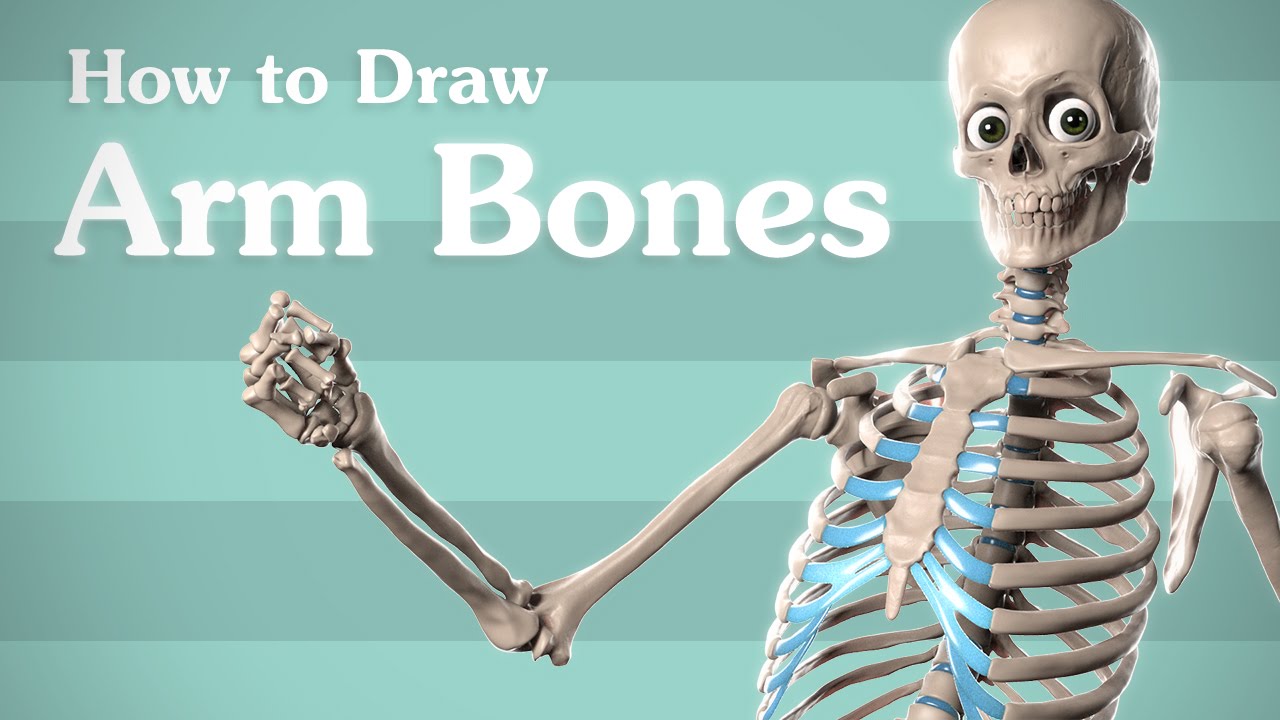In this digitally created, rectangular image, we see a detailed and animated skeleton set against a horizontally-striped green background that alternates between seafoam green and a darker, light forest green. The skeleton is positioned on the right-hand side, leaning slightly to his left (our right). Notably, he has large, expressive eyes with black irises, giving him a happy and excited appearance. Although he has eyeballs, the nose area is missing, emphasizing the skeletal structure.

Prominent at the top left of the image are the words "How to Draw Arm Bones" in white text, highlighting the instructional nature of the illustration. The skeleton’s arm is outstretched and bent at the elbow, drawing attention to the detailed rendering of the arm bones. His chest area is particularly notable for its blue cartilage connecting the ribs to the sternum, contrasting with the otherwise white bones and illustrating anatomical details.

This image, which could be a book cover or educational poster, expertly blends anatomical accuracy with a touch of animated charm, ideal for instructional purposes.